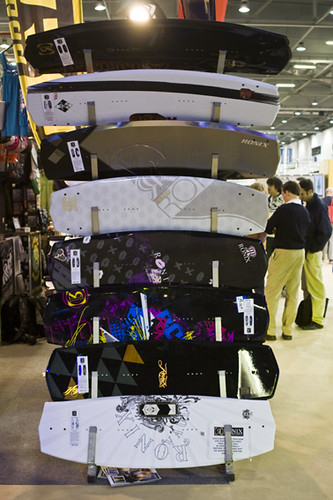The image depicts a colorful display within a sporting goods store, showcasing a vertical rack of eight snowboards, each differing in design and color. From top to bottom, the snowboards are: a solid black one; a white one with a black stripe; a gold one with black accents; a white one adorned with a checkered pattern and the letters "R-O"; a black one featuring the text "X-O"; another black one with vibrant neon hues of blue, pink, yellow, and purple; a black snowboard with gold and gray triangles; and a white snowboard at the bottom labeled with the word "R-O-N-I-X". In the background, the store's ambiance includes the faint silhouette of three people, two of whom wear light-colored pants and black sweaters, and one whose head is blurred, showcasing dark hair against a pale complexion. The photograph, clearly taken in a retail environment, may have been intended to highlight the variety of snowboards available in stock.